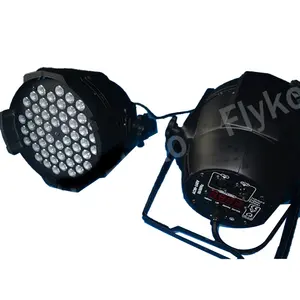This image displays a piece of lighting equipment set against a white background. On the left side, there is a black, cylindrical housing featuring circular LED lights arranged in a honeycomb pattern, with some small beads visible around it. A cable extends from the back of this housing to the right side of the image, which shows the rear view of a similar lighting enclosure. This right section includes a support stand, power cords, and a digital display screen, which is currently turned off. The device has an ink mark with the brand name "FLYKO" and some small, white text likely indicating technical specifications such as voltage. This setup appears to be stage or party lighting equipment.